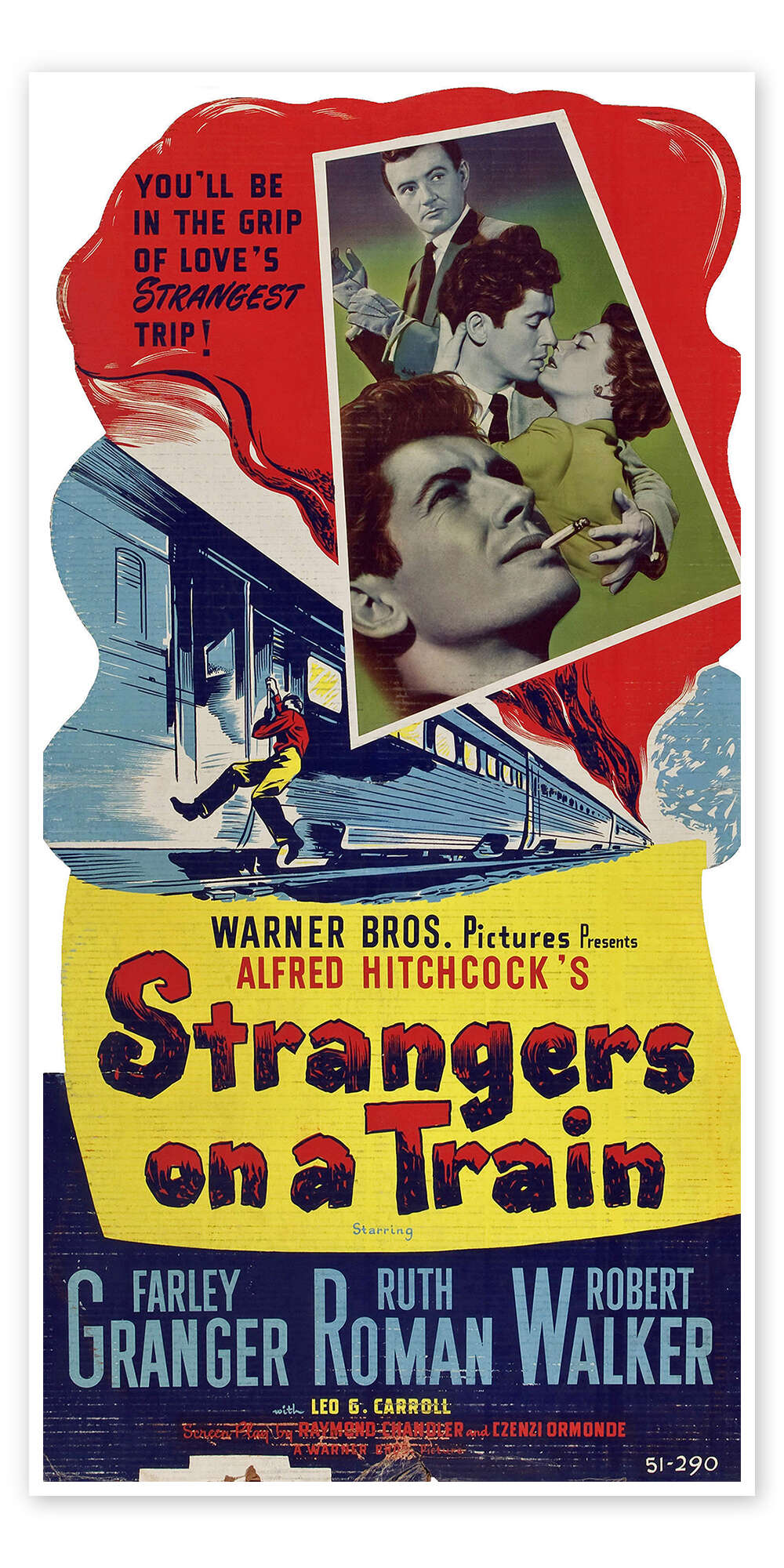The poster for Alfred Hitchcock's "Strangers on a Train" is a striking vertical rectangle, evoking the classic print block style with a retro palette predominantly featuring red, blue, and yellow. Dominating the top, a fiery red area bursts from the roof of a train, adorned with black text proclaiming, "You'll be in the grip of love's strangest trip." This section also showcases black-and-white headshots of the film’s stars, set against a light green backdrop. 

The centerpiece of the poster features a dynamic illustration of a blue train in motion, with a man in a red top and yellow pants dramatically hanging from its side. Beneath this action scene, a bright yellow strip bears the blue text, "Warner Brothers Pictures Presents," followed by the film title in red, "Alfred Hitchcock's Strangers on a Train."

The lower portion transitions to a dark blue background with light blue text listing the main actors: Farley Granger, Ruth Roman, and Robert Walker. Additionally, there are white-framed scenes depicting key moments, including a mysterious man putting on a glove, a man smoking a cigarette, and an intimate moment of a man about to kiss a woman. Subtle white text at the bottom reads the poster number, "51-290," adding a touch of authenticity to this vintage cinematic artwork.